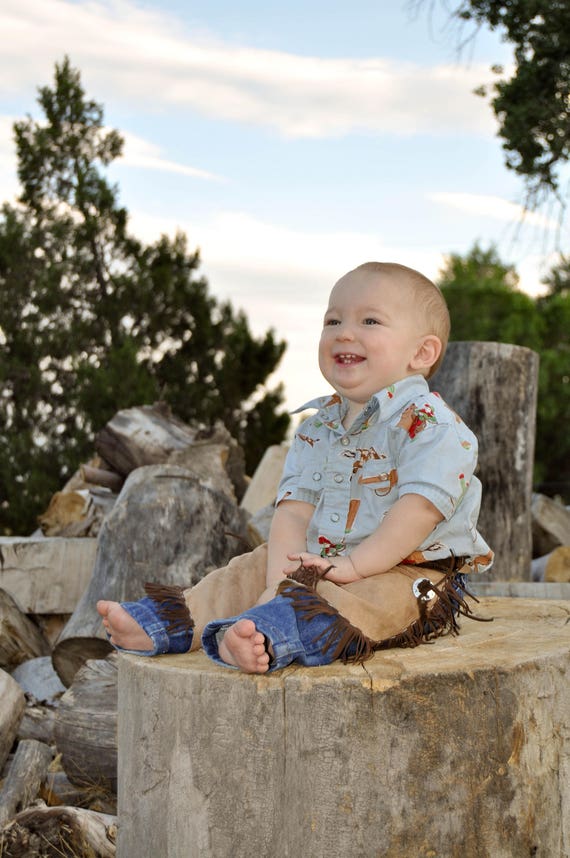In the picturesque outdoor setting of this photograph, a young Caucasian boy, somewhere between baby and toddler age, is captured sitting atop a large, light grayish-brown tree stump. The background features a serene blue sky adorned with a small band of fluffy white clouds, a few tall trees, and a pile of logs stacked together, creating a rustic, natural ambiance. The child, dressed in a light blue button-up blouse adorned with beige and clay-colored cowboy designs, blue jeans, and beige chaps with dark brown leather fringe, sits barefoot, facing the camera yet looking off to the left side of the image. He has short, light brown hair, blue eyes, and an adorably wide smile that reveals several of his teeth, indicating he almost has a full set. This charmingly detailed scene suggests it is part of a photo shoot, likely capturing the innocence and joy of childhood.